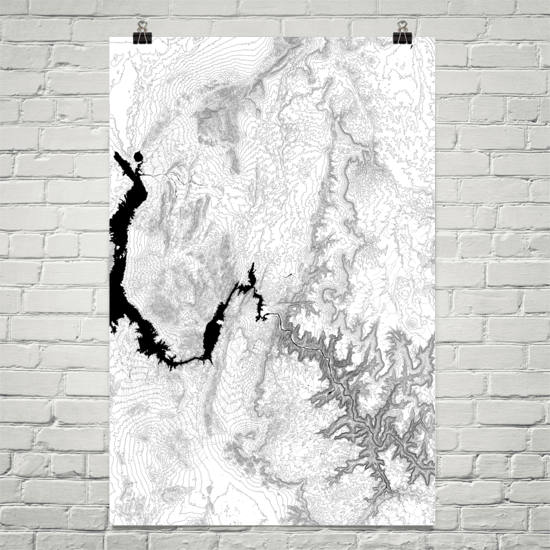A square image, approximately four inches by four inches, depicts a detailed drawing pinned to an off-white, light gray-painted brick wall. The drawing, attached using two black binder clips, presents a top-down view resembling a geographical map. The map features intricate lines and grids drawn using gray pencil and black ink, representing rivers, mountainous terrain, and valleys. A significant river starts in the upper left corner, painted in black ink, and transitions to a darker gray as it flows towards the lower right. The dark and light variations within the drawing highlight different elevations and water bodies. The composition is devoid of roads but rich in natural geographical details, emphasizing the natural waterways and topographical contours.